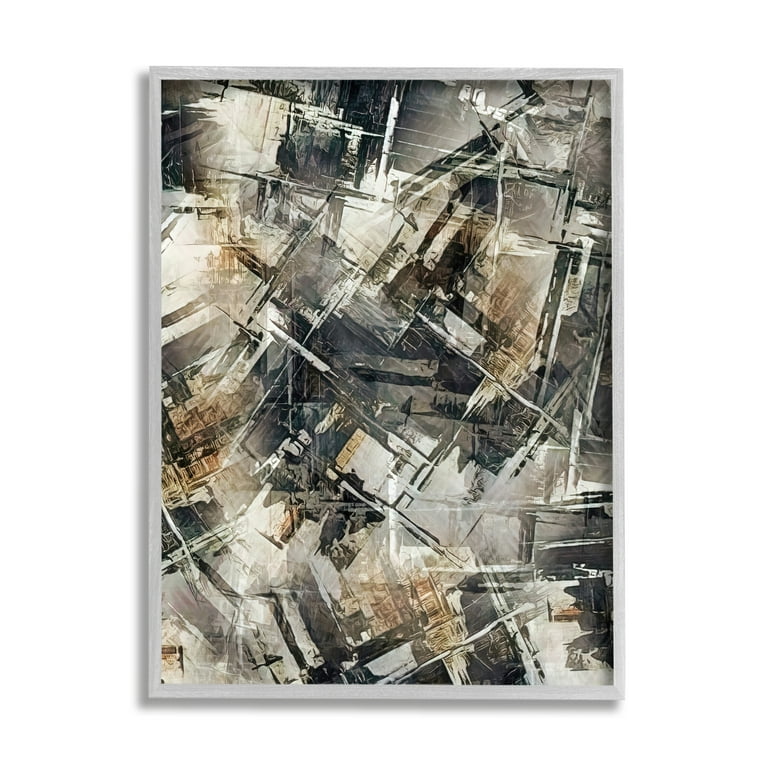The photograph features a painting edited to appear as if floating in an empty white void, emphasizing the clean, featureless background. The artwork is encased in a thin, silver frame that subtly outlines all four edges—top, bottom, left, and right. This abstract painting likely represents a replica or print and is rich in geometric and abstract shapes. It predominantly uses a palette of white, black, and a tannish brown, complemented by grid-like squares and lines in black, white, and tan. The intricate design is reminiscent of a collage of cityscapes, buildings, and shops, with each element appearing slanted and tilted, resulting in an effect akin to multiple transparent layers of city photographs stacked upon one another. The sharp lines and random patterns contribute to the complexity of this visually stimulating piece, devoid of any single, cohesive image, yet evocative of an urban reflection under daylight.